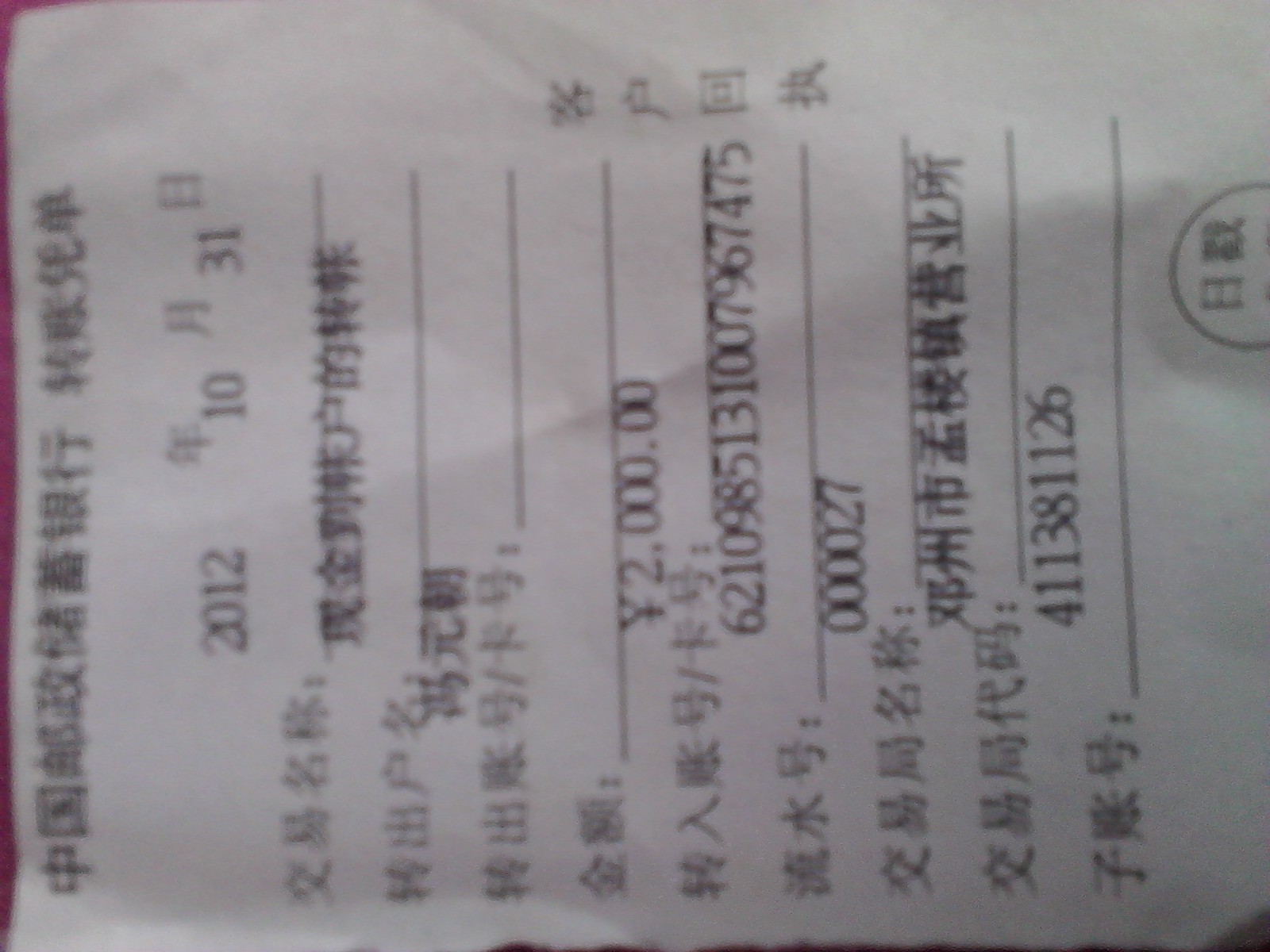This is a high-resolution color photograph featuring a vintage register receipt, printed on traditional register paper. The receipt dominates the frame and is oriented sideways, necessitating a head tilt for proper reading. Inscribed in what appears to be either Chinese or Japanese, the language renders a full translation elusive. However, prominently displayed at the very top is the date "October 31st, 2012," marking this receipt as nearly a decade old. The receipt is densely populated with numbers, indicative of multiple purchases, each item detailed in the foreign script.